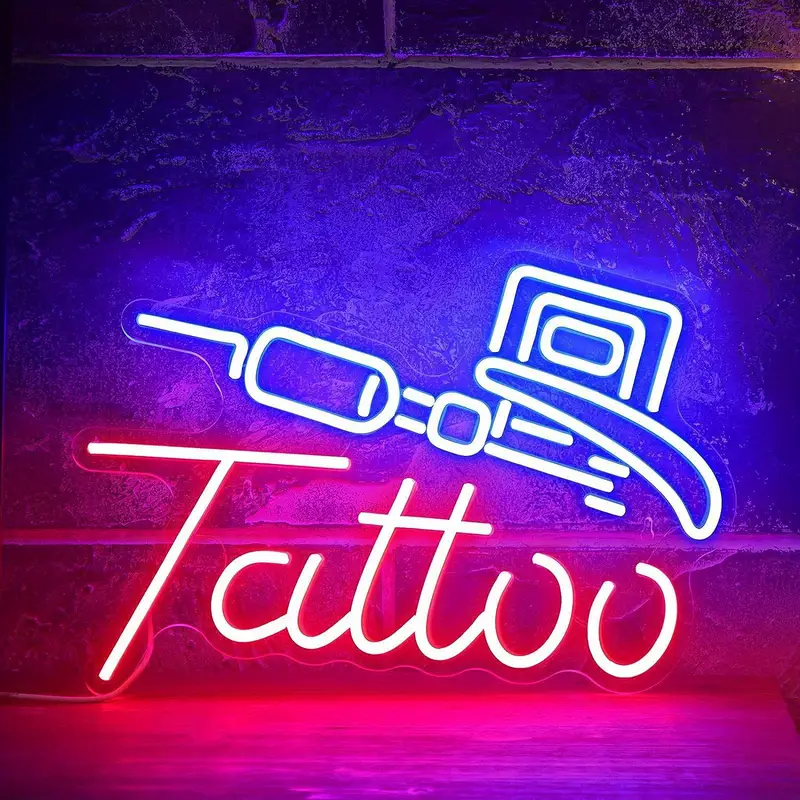The image is a photograph of a visually striking LED sign designed to look like a vintage neon sign. The square-format LED sign features a clear translucent background and is USB-powered for low energy consumption. The bottom section of the sign displays the word "TATTOO" spelled out in glowing white neon-style tubes against a red background. Above the word is an abstract representation of an instrument used by tattoo artists, emitting a blue light. This instrument is positioned at an angle, with its handle pointing toward the right side of the image. The entire composition appears to be leaning against a stone wall, partially illuminated by the vibrant lights of the sign, which enhances its vintage aesthetic.